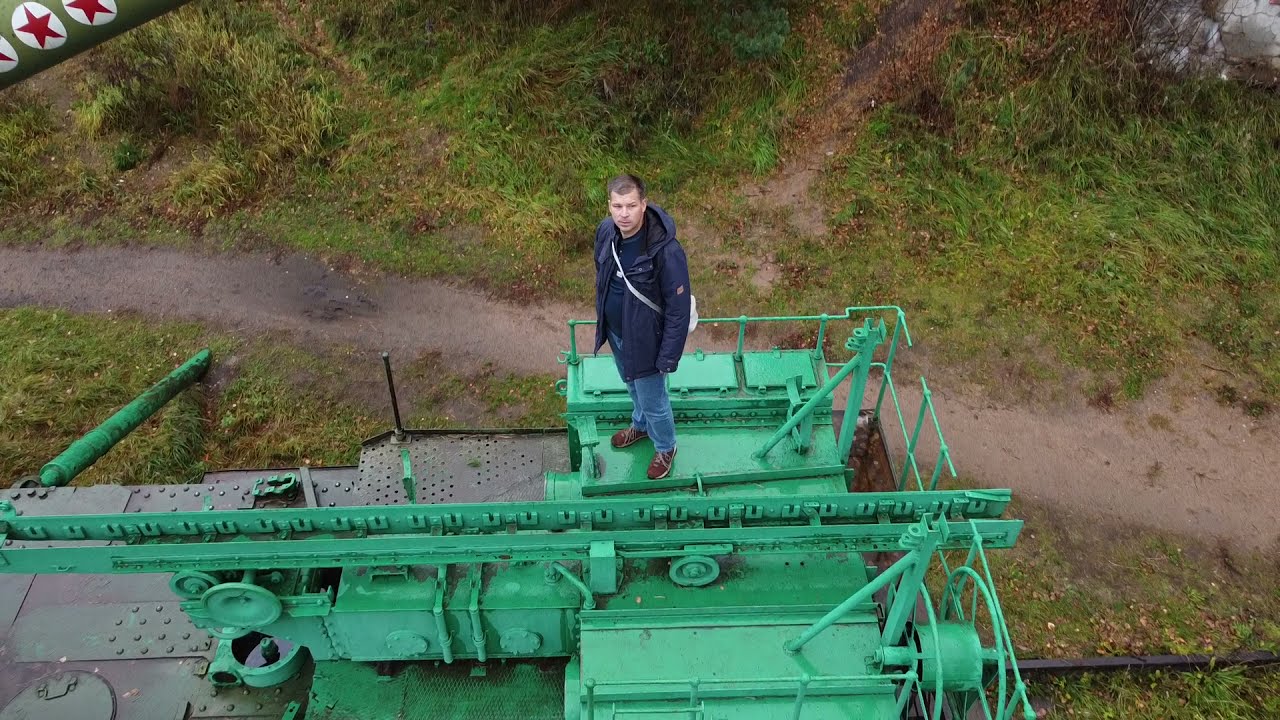In this vivid landscape-oriented photograph taken from an aerial perspective, a man stands at the center of the image on an industrial machine painted a bright, vibrant Kelly green color. This metal equipment, adorned with various pipes, fittings, and wheels, appears to be old military or industrial machinery. Protruding poles stabilize the structure. In the background, a green grassy hillside slopes gently down to meet a dirt path that horizontally bisects the photo.

The man, presumably around 35 to 40 years old, has short dark hair and wears blue jeans, a navy blue hooded jacket over a coat, and brown sneakers. A backpack strap slings across his right shoulder. He looks directly up at the aerial camera with a neutral expression.

In the top left corner, objects with a gray background feature white circles containing red stars, enhancing the military feel. No text is present in the image, and the style is strikingly photorealistic. The setting is vivid and detailed, emphasizing the machine and the man's presence within this lush, open environment.